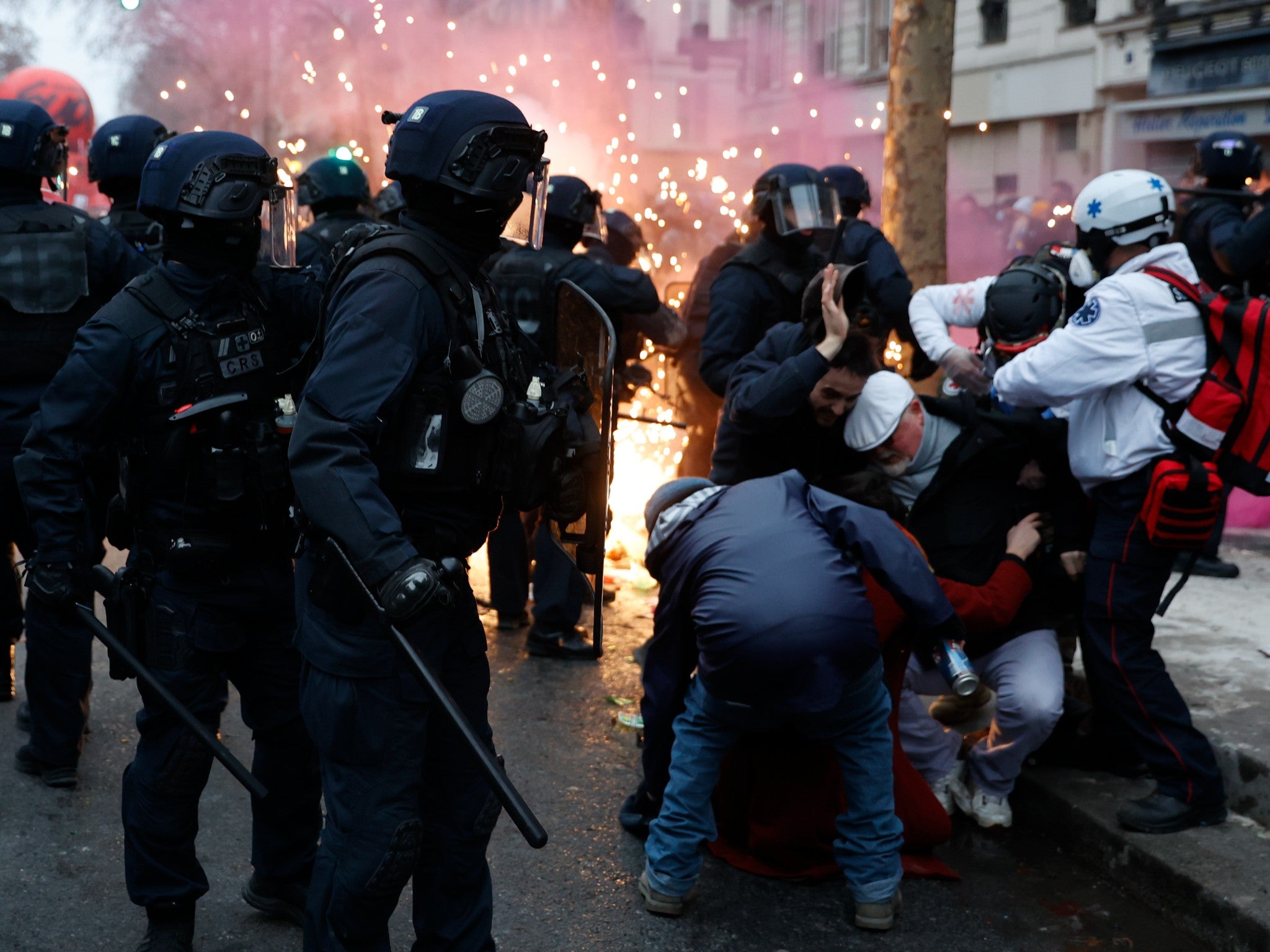This detailed photograph captures a chaotic street riot in an urban area, seemingly in the late afternoon under a cloudy sky. Dominating the left side, numerous police officers clad in black uniforms, riot shields, helmets, and batons are positioned, their protective gear making them appear ready for intense confrontation. To the right, several civilians, including some who might be medics distinguished by their white jackets and red backpacks, seem to be either being attended to by the police or are in distress. The background reveals a tumultuous scene with visible sparks, possibly from fireworks or an ongoing fire, casting light on thick smoke rising into the air. Amidst the tension, many police officers appear alert and somewhat startled, scanning their surroundings. The backdrop of the image reveals a line of buildings, marking the cityscape that has been engulfed in the unrest.